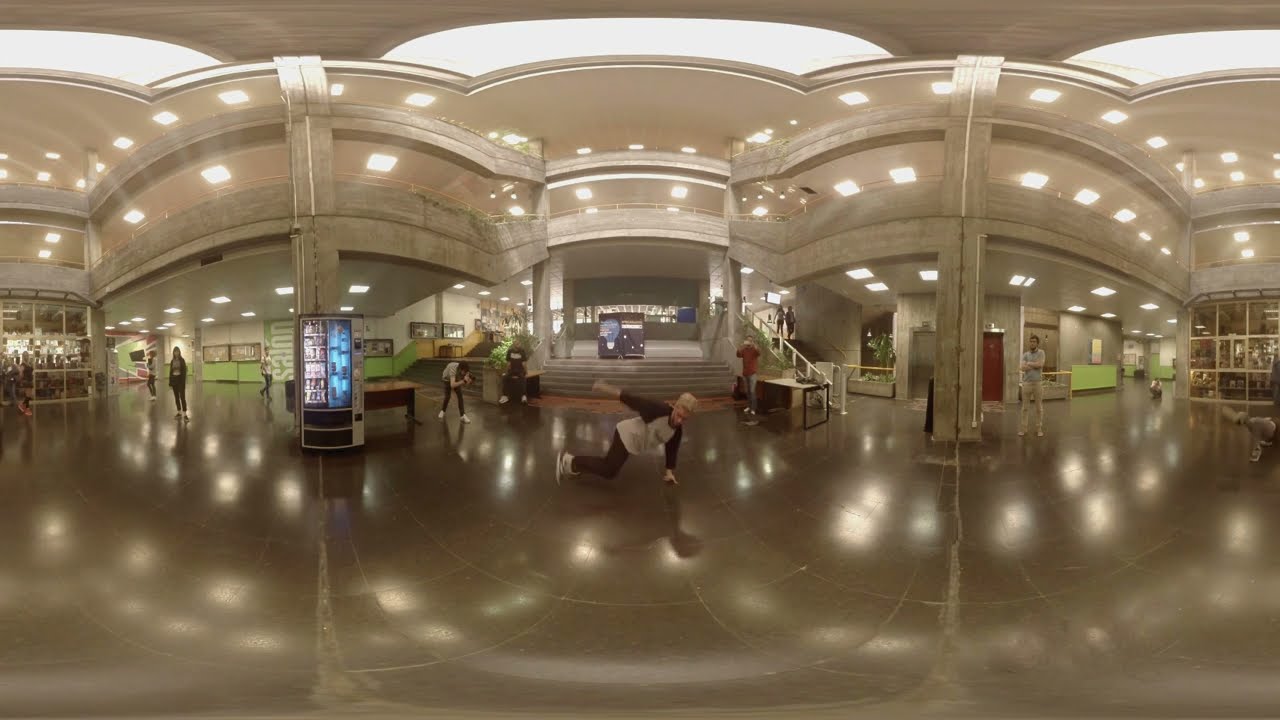In a vibrant public space that appears to be a school or similar institution, the scene captures a dynamic moment centered around a break dancer who is poised just above the ground, skillfully balancing on one hand with a bent knee positioned at an angle. The floor, a shiny dark gray, reflects the overhead spotlights, adding to the energy of the scene. To the left of the break dancer, a photographer is bent forward, intently capturing the action, suggesting a possible commercial or project-related context.

Adjacent to the photographer is a vending machine, which is distinctly split into sections displaying white and blue objects. Further left, a group of people is seen walking past a store, contributing to the bustling atmosphere. On the right side of the break dancer, another person is also engaged in photography, indicating that this might be a coordinated event with multiple perspectives being captured. 

Beyond the immediate activity, a black staircase dominates the background, through which several individuals are descending, emphasizing the public and possibly educational nature of the setting. Concrete textures, green painted accents, and various structural elements like tables, stairs, and elevators define the architectural style of the area, which overall has a white-ish hue. This intricate blend of architectural details and human activity creates a vivid and engaging snapshot of a lively communal environment.